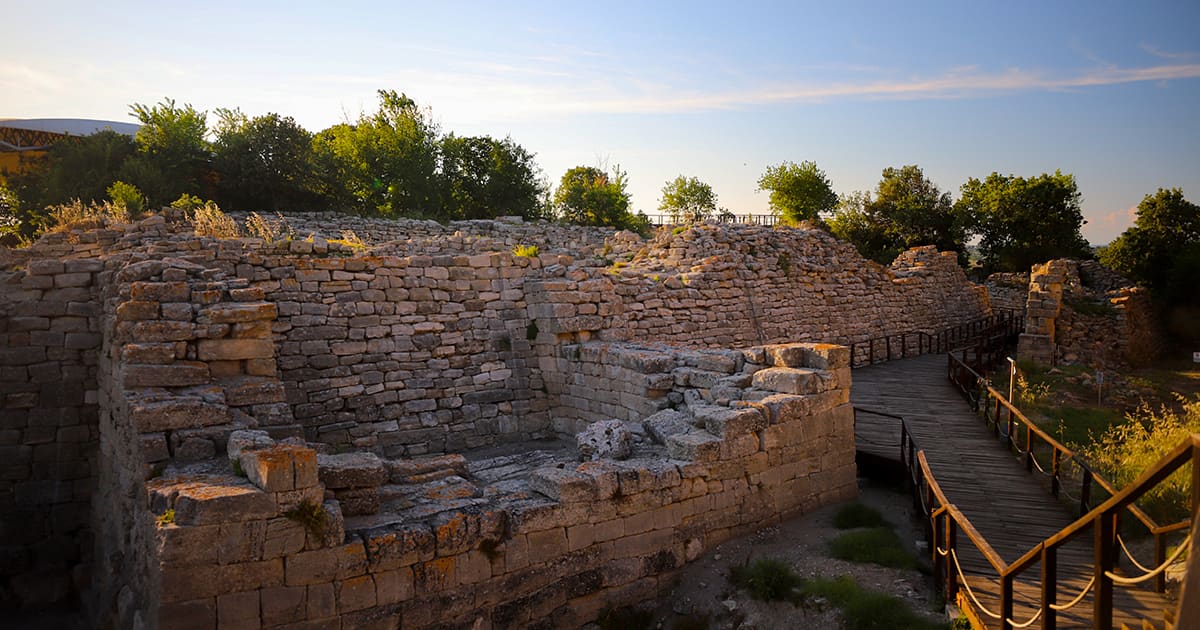The image depicts an ancient archaeological site characterized by its blend of brick, clay, and terracotta-colored stone structures. Central to the composition is a partially preserved building with three prominent walls jutting out from a longer wall, hinting at the remnants of an old stone building. The walls, which appear to be made of stone bricks, vary in completeness, with the front one partially intact and the side walls about three-fourths preserved. 

Greenery, including trees and lush bushes, adorns the ridge on top of the longer wall in the background, adding a touch of natural beauty and contrast to the historical setting. The lower part of the image reveals a carefully constructed wooden walkway on the right side, complete with rope-draped railings, designed to guide modern visitors through the site. This walkway, featuring black railings with rope threaded through them, descends via wooden stairs and winds through the archaeological area, encircling the brick walls and continuing along the length of the site. The path is flanked by grass on either side, contributing to the verdant and serene atmosphere against a backdrop of a clear blue sky with a solitary, horizontal cloud streaking across it.